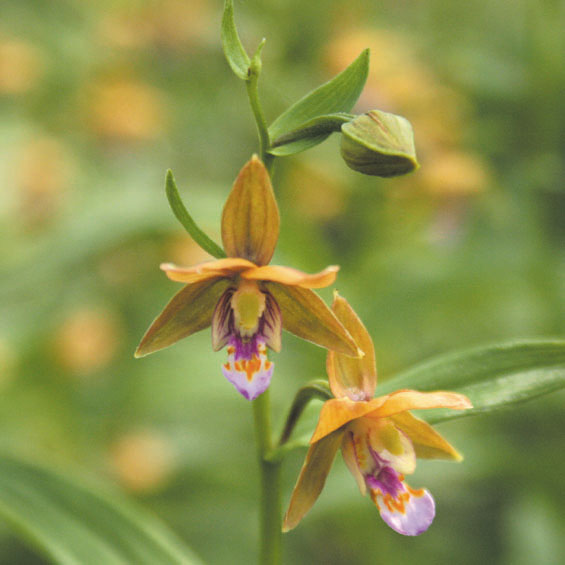This is a detailed close-up image of two yellow flowers with vibrant purple and orange hues emanating from their centers. The flowers are part of a green plant that winds its way up in a wavy manner. One flower bud is prominently featured, suggesting it is about to bloom soon. Surrounding the focal flowers, there are multiple green leaves, including a thicker leaf in the bottom left corner that is slightly less blurred. The background is filled with more of these yellow and purple flowers, but they appear blurred, indicating they are farther away. This image, likely taken in spring, captures various stages of bloom, with green leaves interspersed throughout the background, adding to the lush, verdant ambiance.